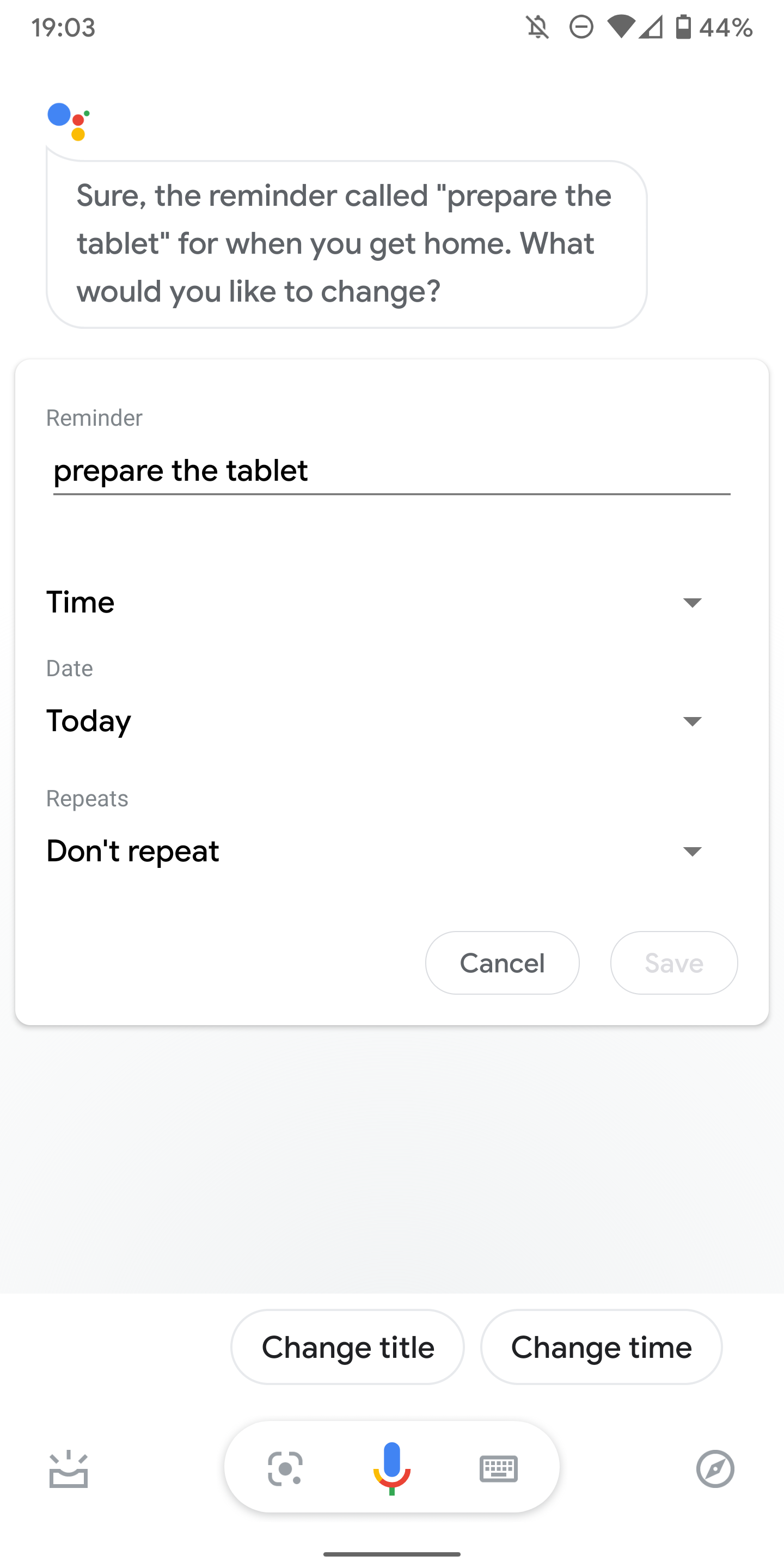This vertical, portrait-style screenshot captures the reminder feature on a Google Assistant interface. The phone's status bar at the top displays the time as 19:03, with the alarm currently turned off. The indicators show a full Wi-Fi signal, a partial cellular service bar, and a 44% battery level.

Beneath the status bar, Google Assistant confirms the creation of a reminder with the message: "Sure, a reminder called 'Prepare the tablet' for when you get home. What would you like to change?" Below this message is a pop-up window providing various options to modify the reminder.

The reminder is titled "Prepare the tablet" and is scheduled for "today" without any repetition. Users can interact with "Cancel" and "Save" buttons situated below these details. At the bottom of the screen, additional buttons are available for "Change title," "Change time," a voice input, a keyboard input, a photo search, and a location setting.

The entire interface is presented with a clean white background and contrasting black text, emphasizing the options available for adjusting the existing reminder within the Google Assistant ecosystem.